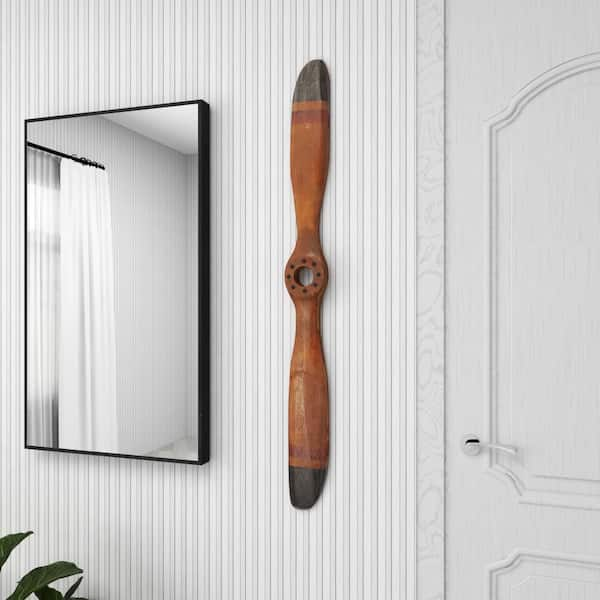This image portrays a meticulously designed white room that exhibits a mix of modern and vintage elements. The room features vertical striped white wallpaper, contributing to a textured yet monochromatic aesthetic. On the right side, a closed white door displays typical oblong engravings and a handle instead of a knob. To the left, a black-framed mirror reflects another part of the room, revealing a window adorned with white floor-length curtains on a black curtain rod. Notably, between the mirror and the door, a vintage wooden propeller blade with black-tipped ends is mounted vertically on the wall, injecting a touch of rustic charm. Adding a dash of vibrant color, a dark green house plant peeks from the bottom left corner, juxtaposed against the predominantly white setting. The elements of brown, black, and green from the propeller and the plant stand out distinctly in this otherwise monochromatic room, creating a balanced and visually appealing space.